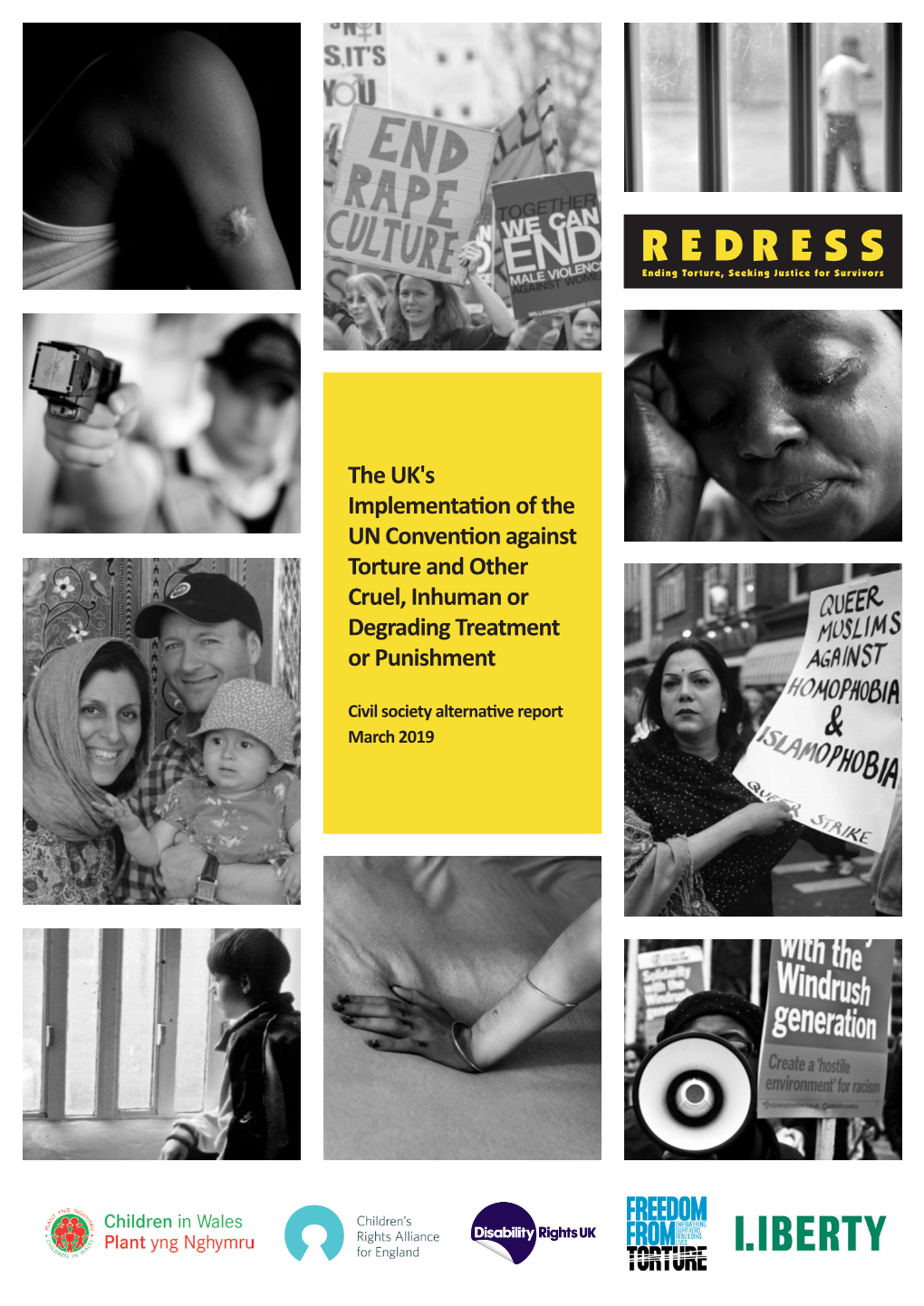The image is a detailed vertical screenshot, likely taken from a website or an email viewed on a phone, depicting a human rights campaign. It is an ad composed of approximately 12 images arranged in a collage style, varying in size and shape, including squares and rectangles.

From top to bottom and left to right, the first image is a black and white photograph of an arm showing visible signs of abuse, including bruises and a scar. Adjacent to this is an image capturing a protest; one sign reads "End Rape Culture" while another says "We Can End Male Violence," held by female protesters.

To the left is an image with the text "Redress: End the Torture, Seek Justice for Survivors," showing a figure behind bars with the word "Redress" prominently displayed beneath it. In the bottom row, there is a blurred image of a person with a gun pointed towards them, creating a tense and threatening atmosphere. Another image depicts what appears to be an immigrant family, adding to the emotional gravitas of the campaign.

At the center of the collage, bold text announces "The UK's Implementation of the UN Convention Against Torture and Other Cruel, Inhuman, or Degrading Treatment or Punishment." This is underlined by the title "Equal Society Alternative Report, March 2019."

Several logos of non-profit organizations are aligned at the bottom, representing Children in Wales, the Children's Rights Alliance for England, Disability Rights UK, Freedom from Torture, and Liberty, highlighting the collaborative nature of this significant campaign.

This caption encapsulates the distressing yet powerful visual elements and the international advocacy efforts depicted in this human rights campaign ad.